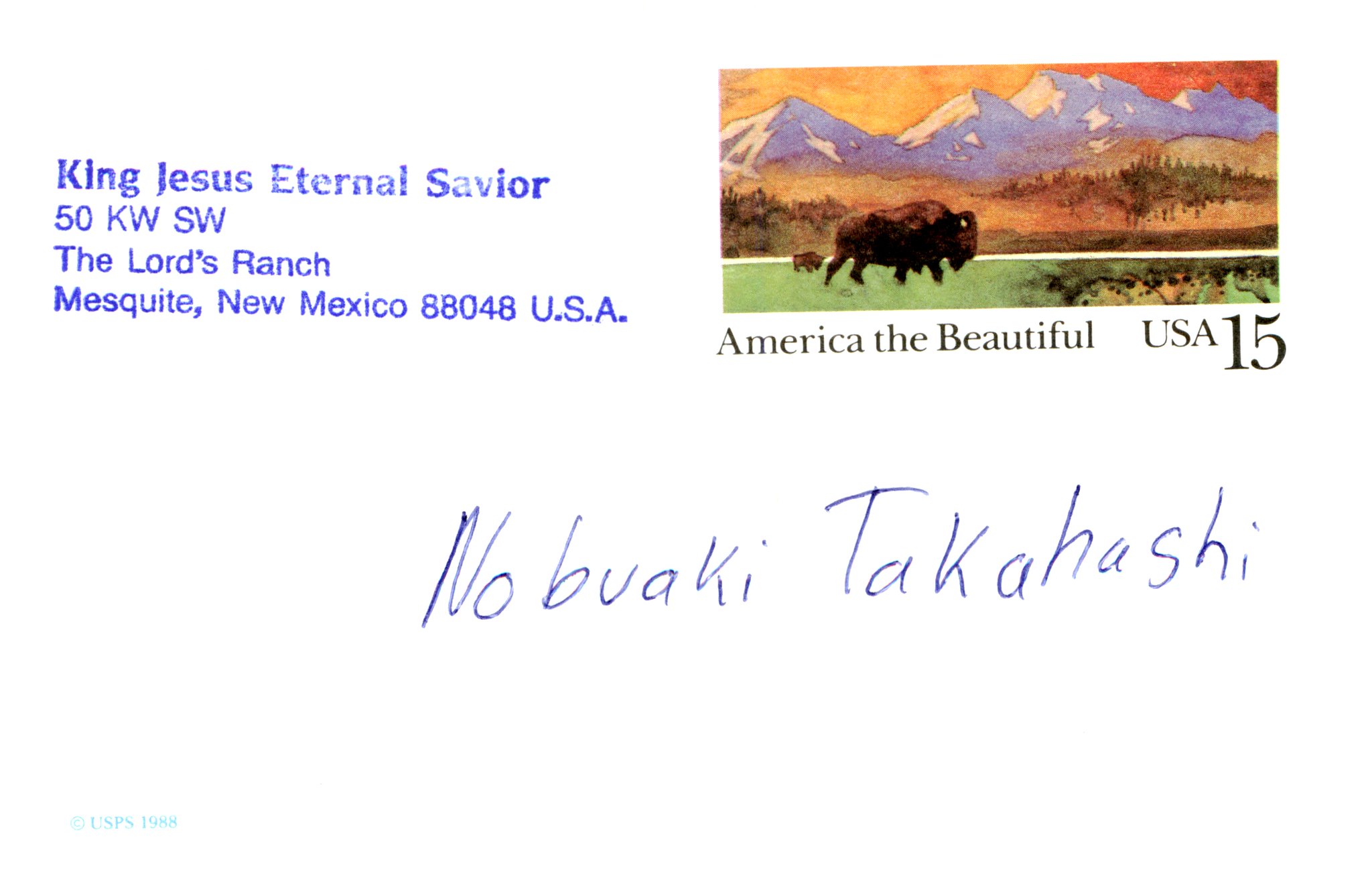A detailed description of the image is as follows:

In this picture, there is an envelope or postcard with a white background. The return address, stamped in blue in the upper left corner, reads: "King Jesus, Eternal Savior, 50 KW Southwest, the Lord's Ranch, Mesquite, New Mexico, 88048, U.S.A." In the upper right corner, there is a postage stamp that features an illustration of an American bison walking across a grassy plain. The scene depicted on the stamp includes a golden-orange sky, white snow-capped mountain peaks in the far background, a sloping hillside leading down to a prairie, and some greenish-brown trees on either side. The foreground shows the bison prominently on the left side, with hints of dirt areas around the grassy field. Below the illustration, the stamp reads "America the Beautiful, USA" in black font, with a large number "15" also in black. The recipient's name, "Nobuaki Takahashi," is written in blue print below the return address.